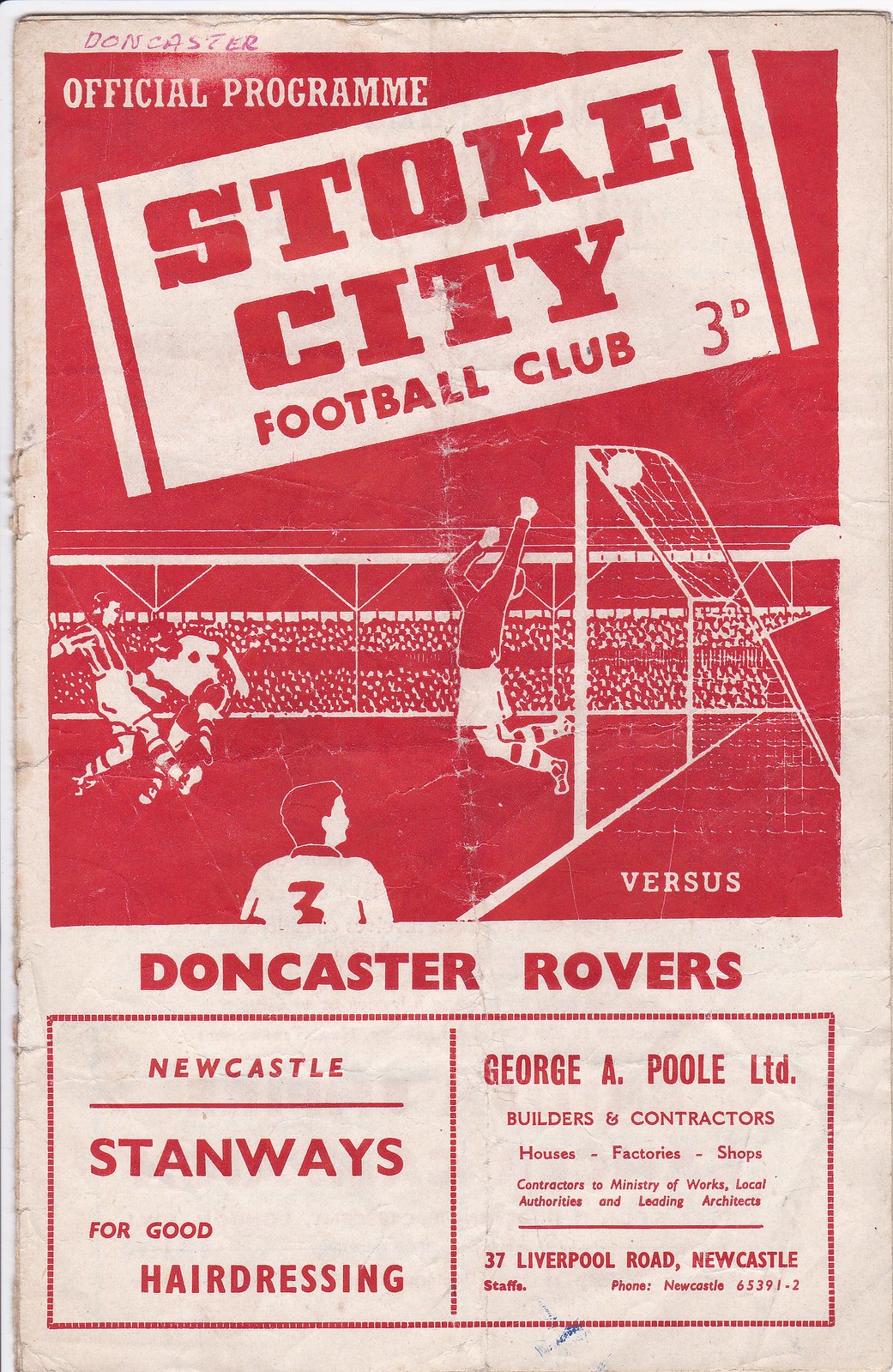This image depicts an official football program for the match between Stoke City Football Club and Doncaster Rovers. The program cover features a vivid red and white illustration of a football scene, rendered in a cartoon-like style. In the foreground, a player attempts to stop a ball from entering the goal, while another player with the number three on their jersey sits to the side. Additional players and a set of stands, drawn in red and black, complete the dynamic scene. At the top, someone has handwritten "Doncaster" in pink pen. The program title, "Official Program, Stoke City Football Club, 3d," is prominently displayed. Advertisements are featured below, including one for Newcastle Stanways for good hairdressing and another for George A. Poole Limited Builders and Contractors, located at 37 Liverpool Road, Newcastle, along with their phone number. The text throughout the program is presented primarily in red and white.